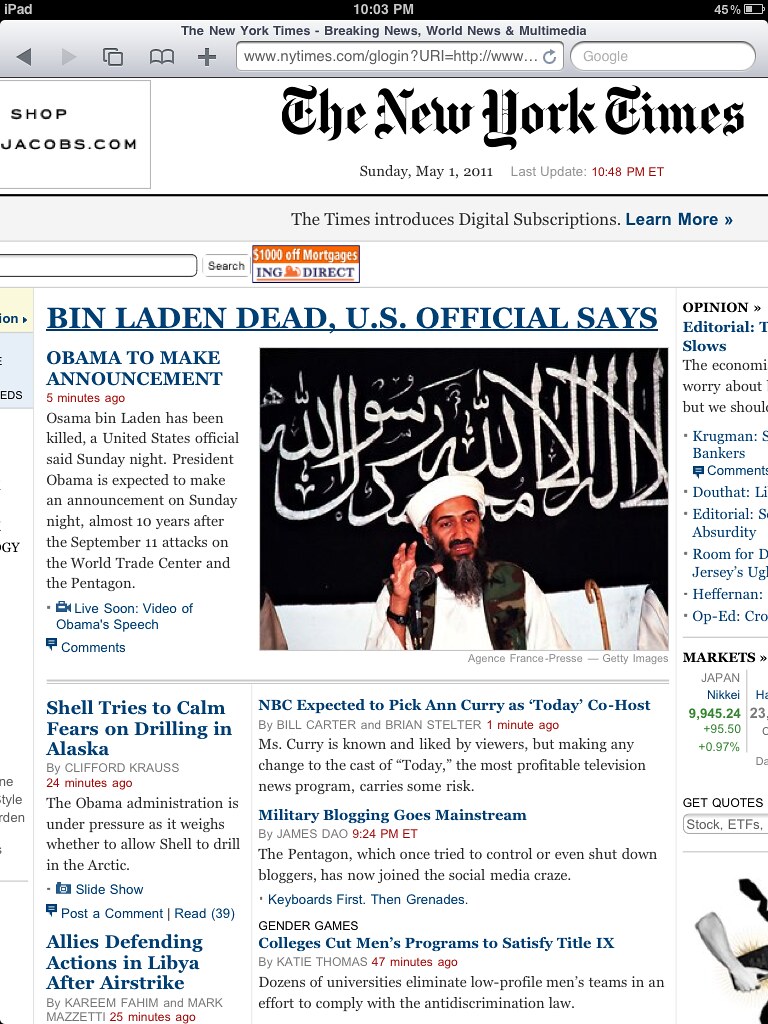This image showcases a New York Times webpage, displayed on an iPad. The iPad is positioned towards the left side of the image. At the top of the screen, the black banner indicates the time as 10:03 p.m., with the battery icon showing 45 percent charge. Below this, the webpage header features sections like Breaking News, World News, and Multimedia. 

The address bar is situated below the header, followed by a Google search bar on the right, and navigation arrows (both left and right) on the left. Additional icons include a page refresh, a bookmark, and a plus sign.

In the main body of the webpage, the publication is identified as the New York Times, with the specific date marked as Sunday, May 1st, 2011, and the last update timestamped at 10:45 p.m. Eastern. A prominent banner informs readers about the introduction of digital subscriptions, with a call to action to 'Learn More.'

The primary article headline reads, "Bin Laden Dead, U.S. Officials Say," accompanied by a photograph of Osama Bin Laden, recognizable with Arabic text behind him, a raised hand, camouflage vest, white head covering, and white garb.

To the right is a section with opinion pieces and market updates, which are partially cut off. Another headline to the left announces, "Obama to Make Announcement Five Minutes Ago," with a related notice underneath for live video coverage of Obama's speech and a comments section.

Further down, an article discusses Shell's efforts to calm fears about drilling in Alaska. Another piece covers allies defending their actions in Libya following an airstrike.

Additionally, there is an article about NBC's expected decision to appoint Ann Curry as the new co-host of "Today," followed by pieces on military blogging mainstreaming and gender issues in colleges cutting men's programs to comply with Title IX.

This detailed depiction encapsulates both the structure and the various segments visible on the New York Times webpage on an iPad.